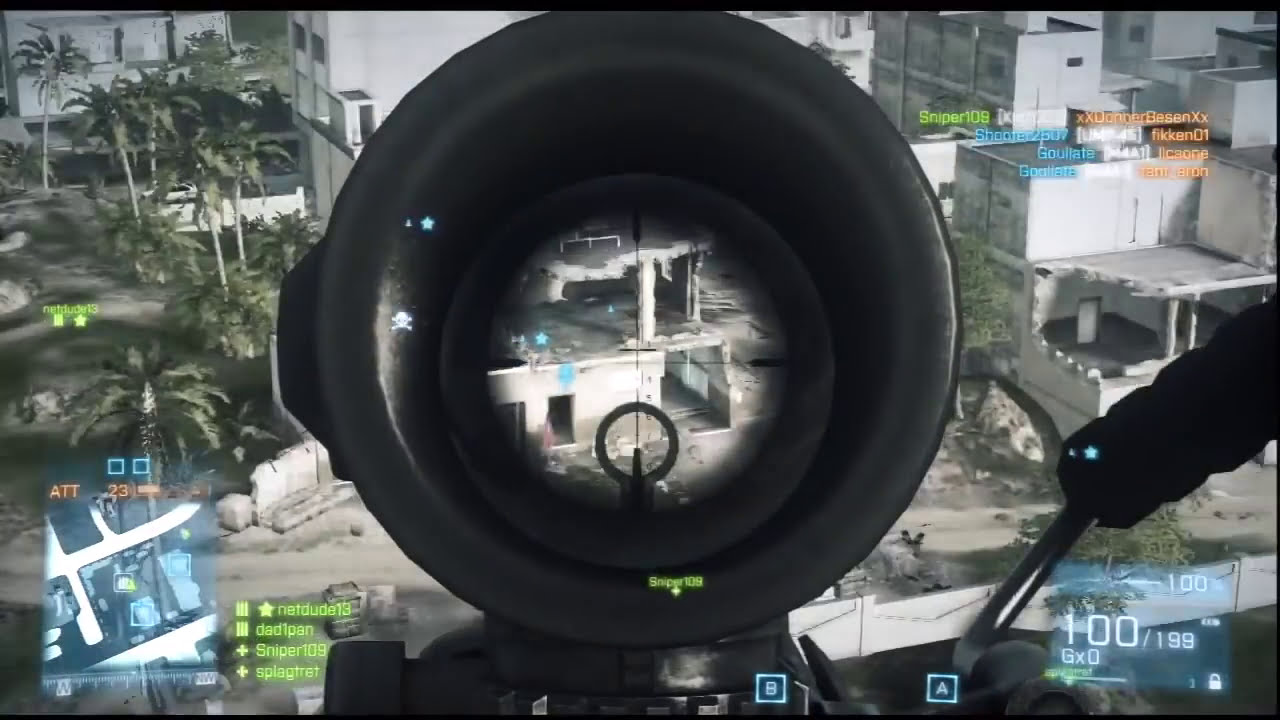The image is a detailed screenshot from a first-person shooter video game, specifically from a Battlefield series game, likely Battlefield 3 or Battlefield 4. The scene features a war-torn warehouse district, characterized by white concrete buildings in varying states of disrepair—some one, two, and three stories tall. Many of these structures have parts blown out, exposing their skeletal frameworks. The district is interspersed with tall green palm trees, providing a stark contrast to the dilapidated surroundings. The player's viewpoint is through the magnified scope of a rifle, focusing on a circular iron sight and a central crosshair. The scope's view zooms into a specific area, showing detailed destruction approximately 50 feet below, while the peripheral view outside the scope reveals more of the devastated cityscape. Various interface elements indicate ammo count and team information, enhancing the immersive experience of the battlefield.